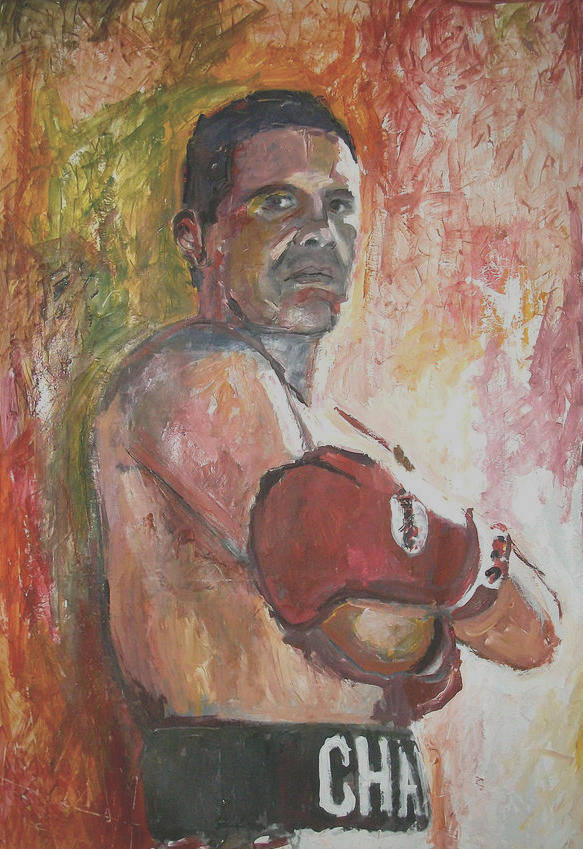This image, likely a watercolor painting, features a serious-looking boxer depicted from the side with his head turned towards the viewer. The boxer has short, dark brown hair and is shirtless, highlighting a slightly discolored, possibly white complexion with brown and gray shading. His left arm is crossed over his right, with his left hand resting just below his right shoulder. Both hands are encased in red boxing gloves with white markings. He is wearing white shorts with a prominent, large black belt around his waist, displaying the letters "C.H.A." 

The background is a vibrant blend of brush strokes. The top left corner is dominated by green tones with touches of orange and white, while the top right corner features a mix of red and white with hints of green. The left side transitions from red and brown to green, and the right side is predominantly white with light brown accents. Overall, the colorful background and detailed portrayal of the boxer create a dynamic and engaging scene.